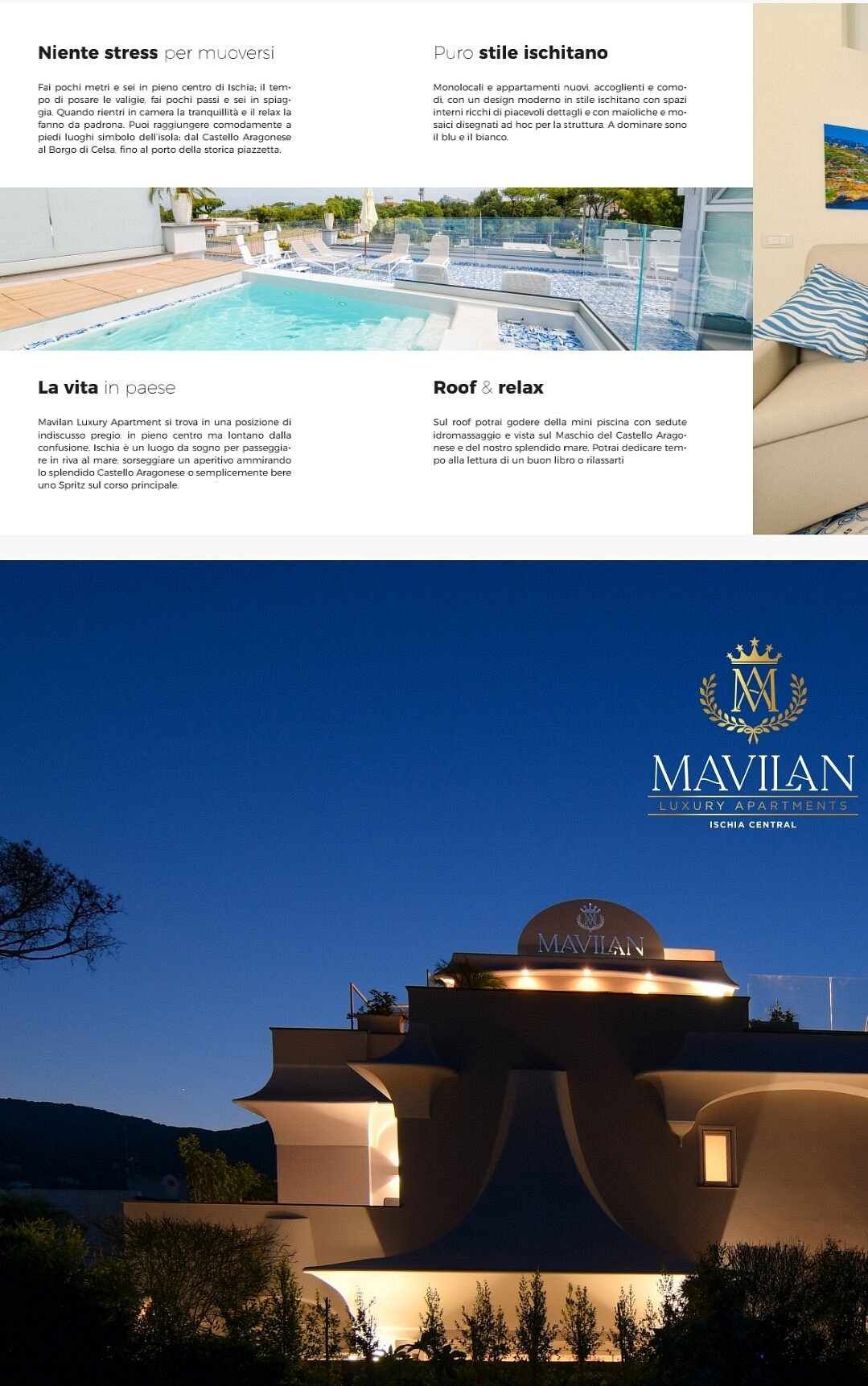The image is a detailed advertisement for Mavalon Luxury Apartments. The top portion showcases a rooftop swimming pool surrounded by glass and a deck, designed for relaxation. This section includes three titled paragraphs of bold text in a foreign language, black on white, accompanying the pool image. The upper right corner features the Mavalon crest and logo in gold with the text "Mavalon Luxury Apartments" beneath. The bottom part displays the exterior of the tan-colored apartment building, with a grand entryway surrounded by trees and a stunning twilight blue sky overhead. A distant mountain range provides a picturesque backdrop. The entire scene suggests a luxurious and serene living environment.